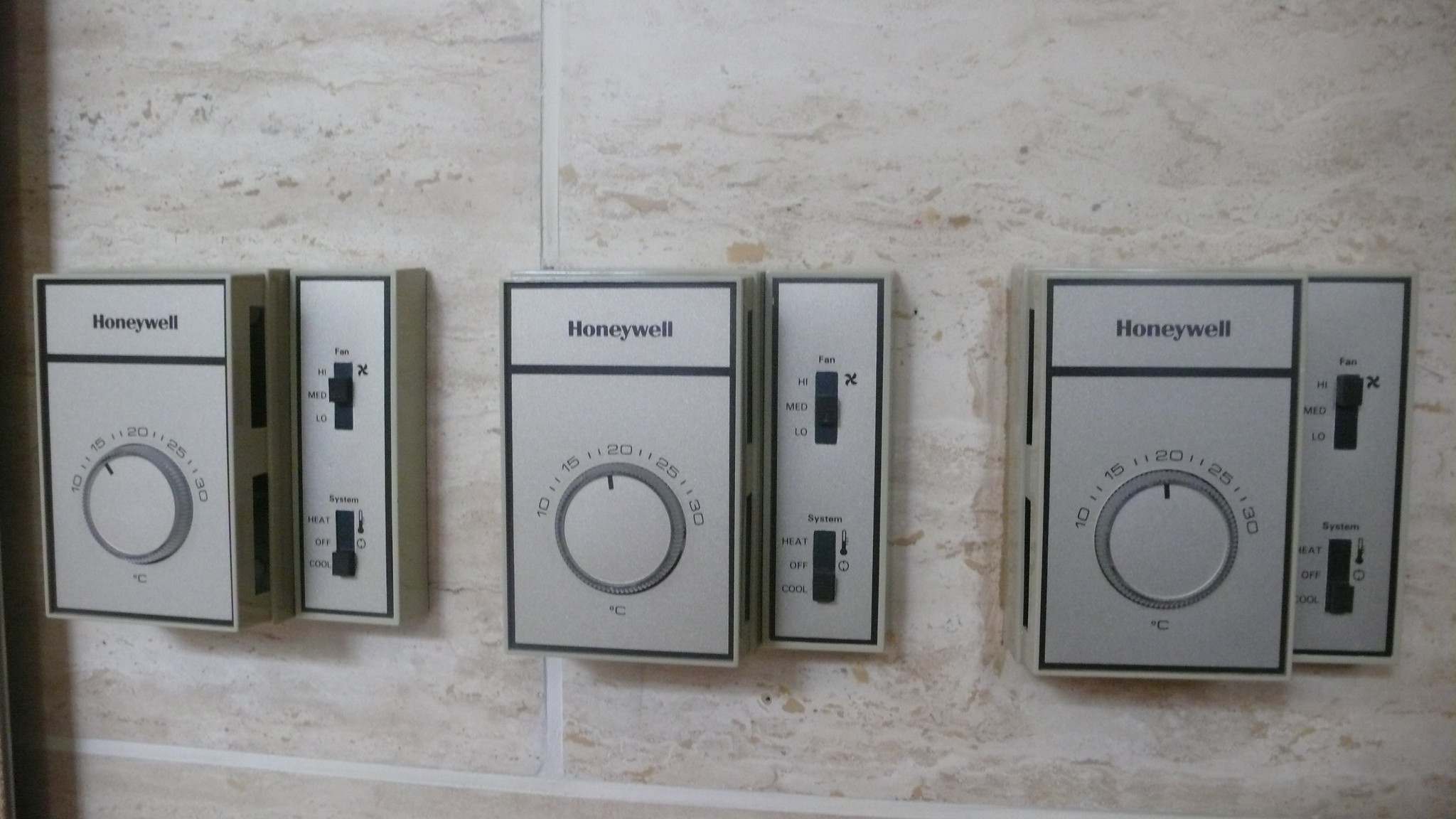This close-up image captures three older-looking Honeywell thermostats affixed to a tiled wall with a beige and speckled texture. The thermostats are arranged vertically in succession and are rectangular with a square-shaped top segment. Each top segment features the Honeywell logo in black. Below the logo, there is a numbered dial with a small black knob for adjusting the temperature, marked in Celsius with increments of 10, 15, 20, 25, and 30 degrees. The bottom sections of the thermostats have a secondary vertical panel with two black switches. The top switch controls the fan settings, labeled 'High,' 'Medium,' and 'Low,' while the bottom switch is for the system settings, offering options for 'Heat,' 'Off,' and 'Cool.' The thermostats are positioned adjacent to each other, each with similar configurations, with one thermostat set to 15 degrees Celsius and another slightly below 20 degrees Celsius.